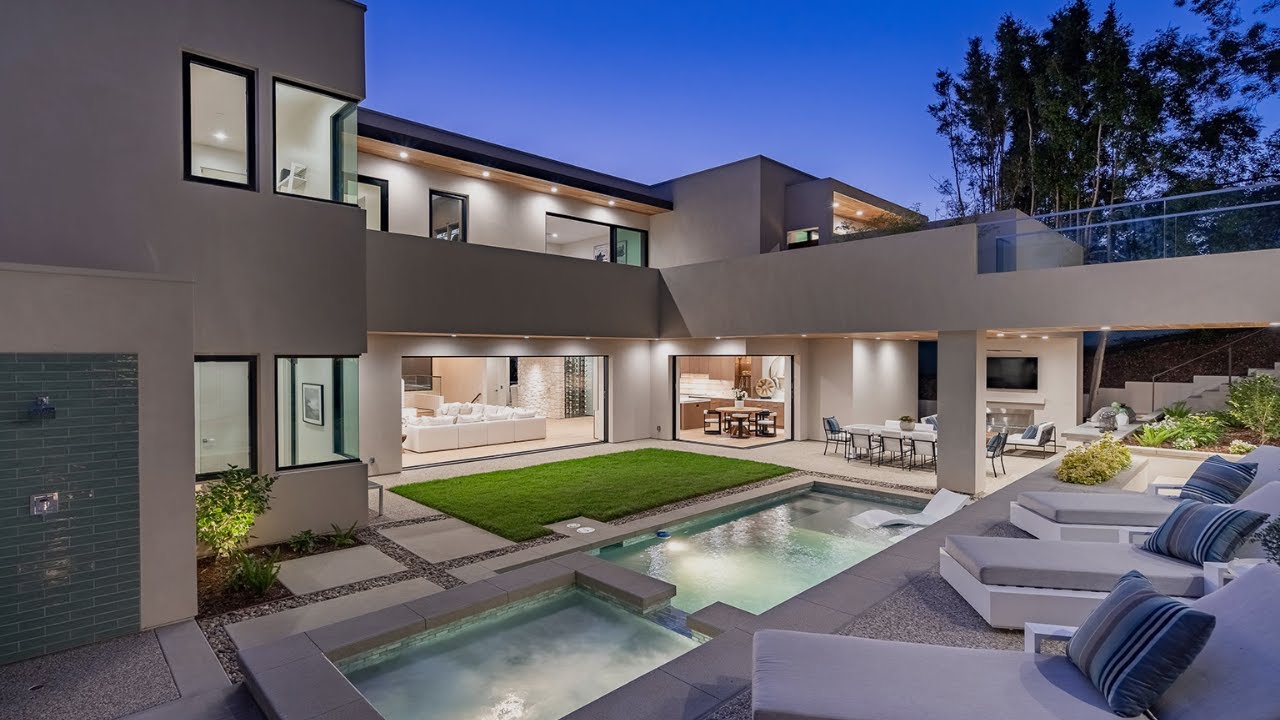The image depicts a luxurious, modern mansion at dusk, set against a deep blue sky. The architecture features clean lines, a predominantly white concrete or stucco surface, and an abundance of large windows. The two-story home is illuminated by exterior lights, which enhance its contemporary design. 

In the foreground, the outdoor area includes three lavishly padded lounge chairs with blue striped pillows, positioned near a small, minimally-sized pool and hot tub. Adjacent to this area is a stone and concrete-paved space with an outdoor shower. The backyard also boasts a rectangular patch of lush green grass.

Beyond the pool, there's a large sliding glass door that opens up to reveal the interior, showcasing a spacious living room with a white couch. To the right is an open-plan kitchen and dining area connected to an additional outdoor dining space under the covered patio, which features a TV and a fireplace. On the second floor, a pathway extends from the right off-screen into the housing area, with lit windows providing a glimpse into the rooms without revealing specific details. Trees frame the right side of the house, adding to the overall affluent and serene ambiance of the scene.